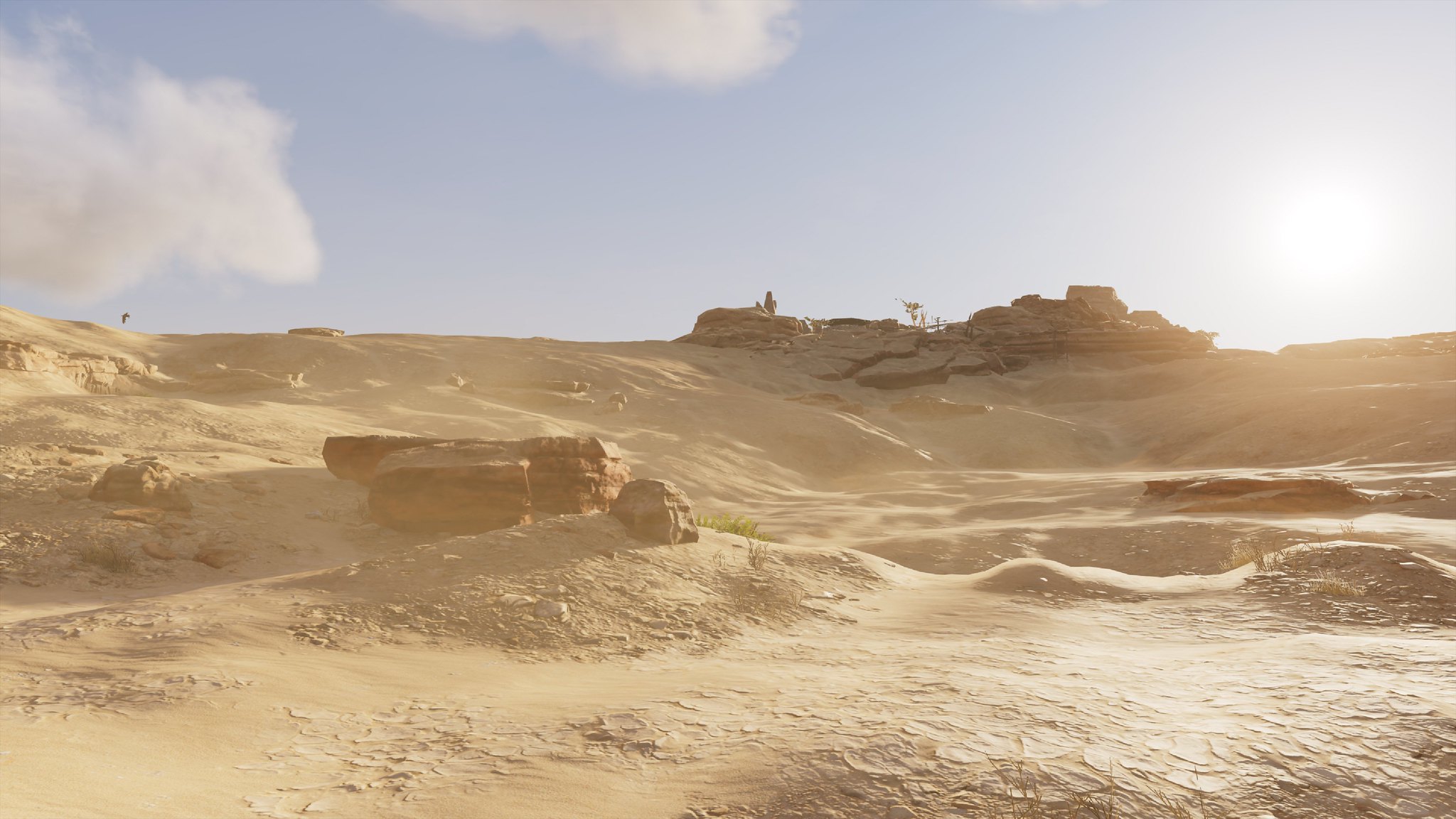This image displays a vast, barren desert landscape with a strikingly uniform light tan ground, which appears parched and cracked from prolonged dryness. The entire background consists of expansive sand dunes accented by sparse rocky outcroppings and boulders, especially noticeable towards the center-left of the frame. In the upper right corner, a bright, blurry white sun casts a harsh light across the area, illuminating the cracked earth below. The sky is a vibrant, clear blue, contrasting sharply with the arid desert below. Two fluffy white clouds drift near the left edge of the image, almost touching the sand dunes. Amongst the desolation, subtle hints of life are visible: a cactus, a few small shrubs, twigs of grass, and perhaps a small bush nestled in a valley between the dunes. In the upper left corner, atop a rocky outcrop, there might be a tree or possibly a person hiking, adding a sense of scale to the otherwise lonely scene.